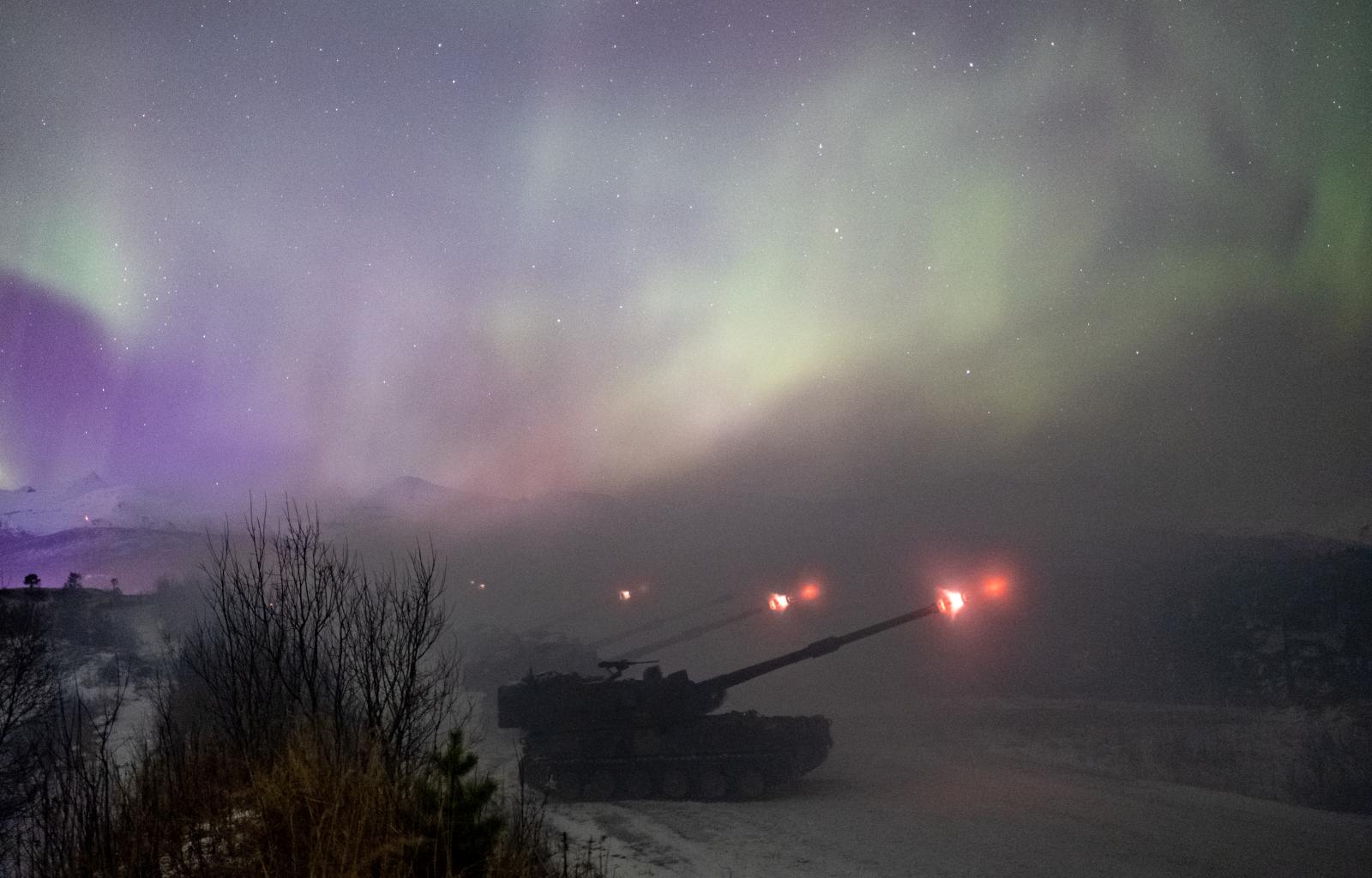Under the vibrant night sky adorned with the shimmering northern lights—displaying hues of purple, green, and streaks of red and orange—a dramatic scene unfolds. In a cold, mountainous landscape blanketed in snow, a line of at least five military tanks is captured in the midst of coordinated action. The tanks' cannons erupt simultaneously, sending bright embers and projectiles into the night, creating a spectacle of light against the darkened, star-studded sky. The distant, snow-covered mountains and sparse vegetation, combined with the ethereal glow of the aurora borealis, enhance the striking visual intensity of this moment. The scene appears to be set in the far northern climate, emphasizing the stark, breathtaking beauty of the natural and the martial harmoniously clashing under the celestial display.